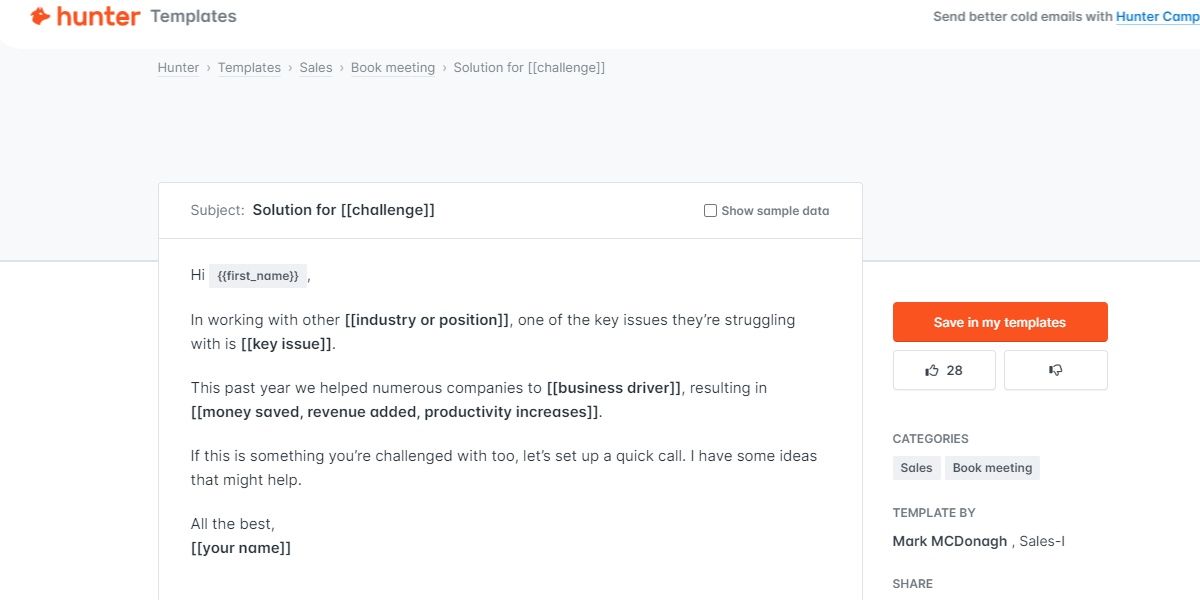The image depicts a screenshot of a template provided by the brand "Hunter," which specializes in creating templates. In the upper left corner, the Hunter brand logo and name are prominently displayed in orange, accompanied by the word "Templates" in gray.

On the upper right, the text reads, "Send Better Cold Emails with Hunter Comp." This is followed by several navigational sections: "Hunter," "Templates," "Sales," "Book Meeting," "Solution for," and "[Challenge]."

Beneath this, the template layout begins with a placeholder for the email "Subject" and repeats "Solution for [Challenge]." On the right, there is an option to "Show Sample Data," with an unchecked box next to it.

The email template reads as follows:
- "Hi, [First Name],
- I’m working with other [Industry or Position]. One of the key issues they’re struggling with is [Key Issue]. This past year, we helped numerous companies to [Business Driver], resulting in [Money Saved, Revenue Added, Productivity Increases]. If this is something you’re challenged with too, let’s set up a quick call. I have some ideas that might help.
- All the best,
- [Your Name].”

On the far right of the template, there is an orange button labeled "Save in My Templates." Below this button, there is a "Thumbs Up" with the number 28 next to it and a "Thumbs Down" with no number. Under these, the categories "Sales" and "Book a Meeting" are listed.

At the bottom, it mentions that this template was created by Mark McDonough, tagged with "Sales-1," and includes a "Share" option.

Overall, the template on the site, Hunter Templates, was crafted by Mark McDonough. There are no additional texts outside the specified content fields.